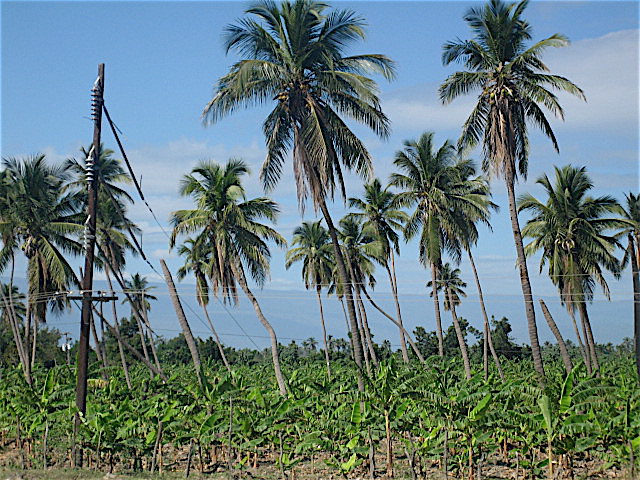The image captures a lush, expansive plantation filled predominantly with palm and coconut trees of varying heights, some towering over 6 meters tall. The scene is bathed in natural sunlight under a partially cloudy sky, with hues ranging from vivid greens of the plants to the blue and white shades of the sky. In the foreground, the green field brims with diverse plants and small coconut trees, while the taller, mature coconut trees stretch towards the background, where the plantation seems endless. Several of these tall trees appear to have been cut, standing as mere stumps. Further in the distance, a large body of water faintly glimmers, adding depth to the scenery. Noticeably, power lines and a pole with silver elements are visible in the front left of the image, hinting at infrastructure within this natural setting. The photo, taken during daytime, is rich with vibrant colors and devoid of any people or vehicles, suggesting a serene and undisturbed landscape. This composition, brimming with tropical flora and enhanced by its bright, sunny weather, hints at a location perhaps overseas, reminiscent of regions like Vietnam.